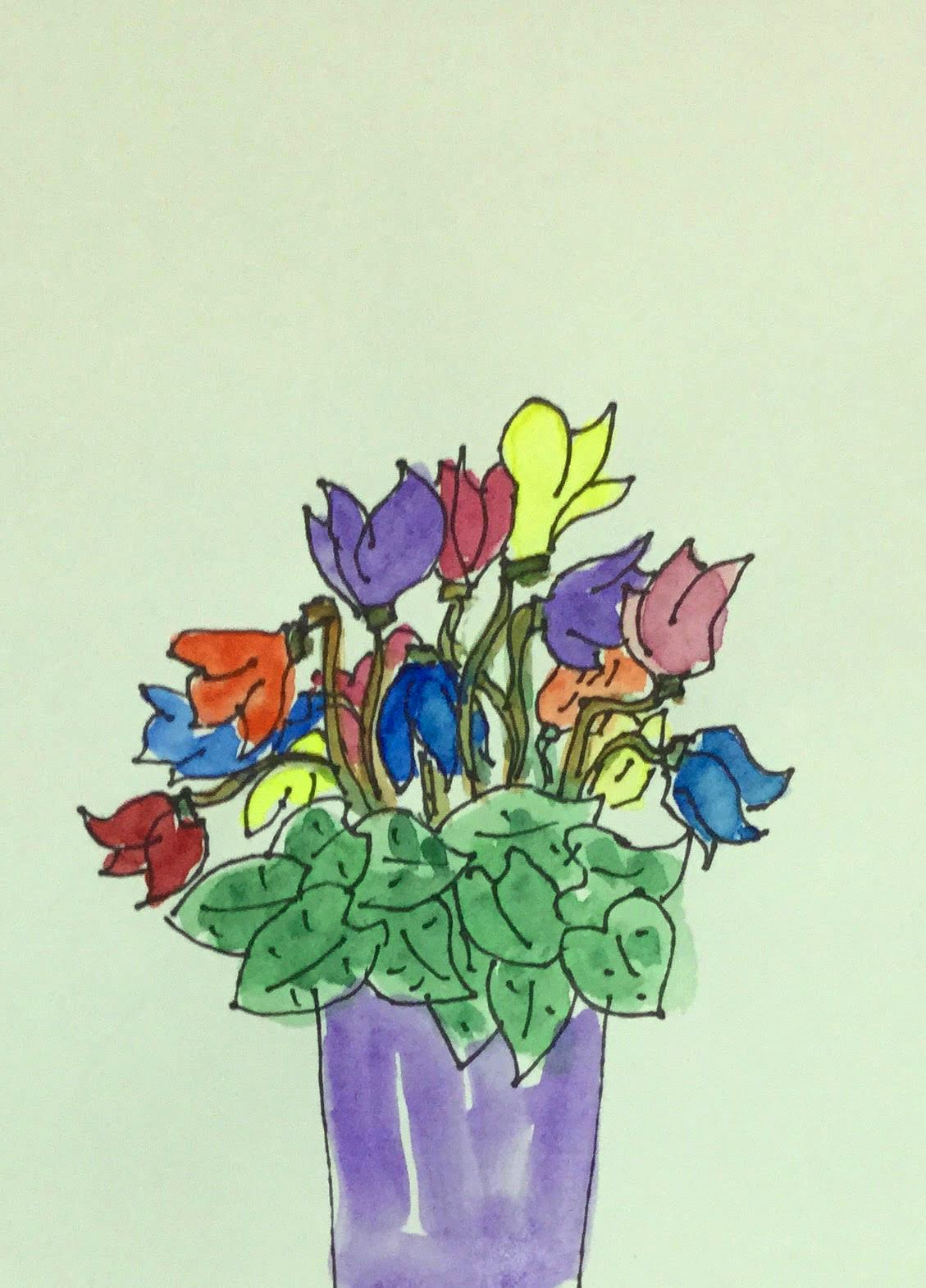This image is a drawing rendered on a very light grayish-green paper. The drawing, situated towards the bottom of the page, features a purple plant pot depicted with broad, simple strokes. The leaves of the plant are sparsely detailed, likely created with black ink, pencil, or marker, and partially filled in with patches of green. The standout feature of this drawing is the assortment of flowers bursting from the plant. These flowers are marked by a vibrant and varied palette, including maroon, sky blue, orange, yellow, royal blue, purple, and lavender, adding a lively and colorful contrast to the subtle background.